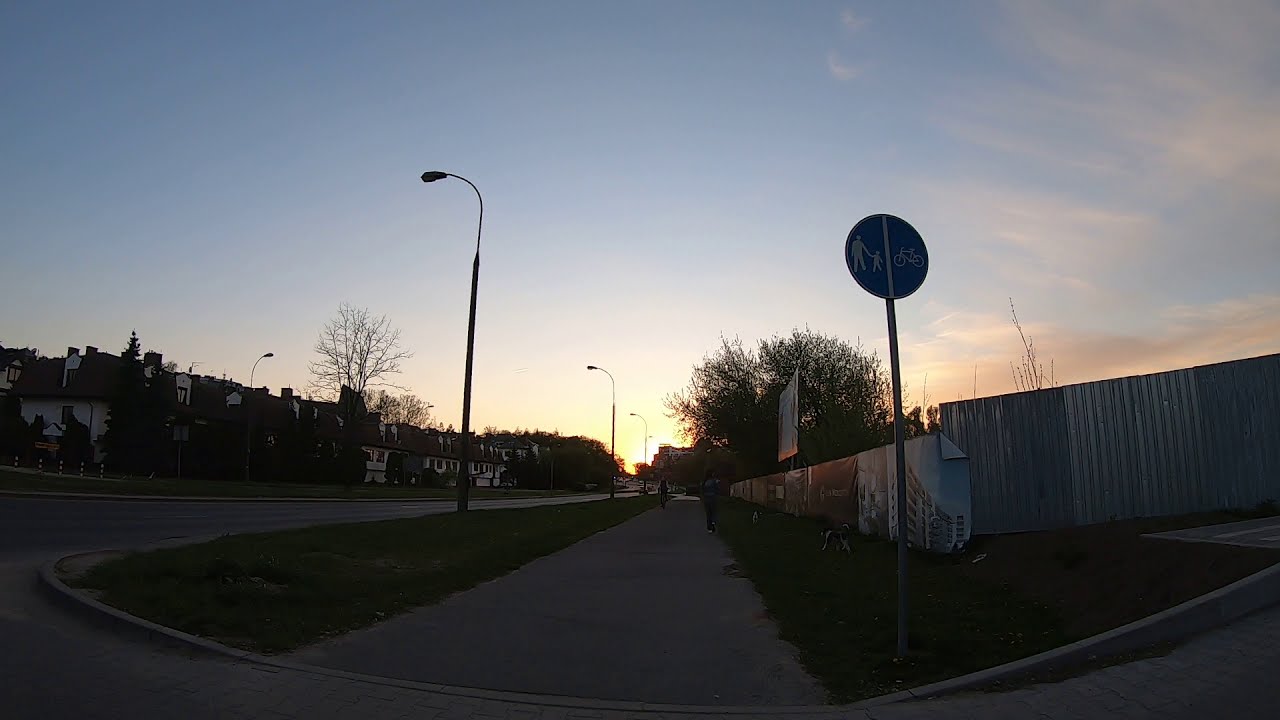In this image taken at dusk, we see a wide sidewalk extending through what appears to be a residential community. The sky, tinged with the soft hues of sunset, features the sun setting directly in the middle of the composition. To the left of the sidewalk, a piece of land with a grassy patch and telephone poles separates the path from the road. On this road, there are no cars, enhancing the tranquil and quiet atmosphere. 

Dominating the foreground is a distinctive circular street sign, bisected vertically into two halves – one side depicting an adult holding a child’s hand, and the other side showcasing a bicycle, indicating that the path is designated for pedestrians and cyclists. The sidewalk, possibly a large walking path, stretches into the distance, where a few people and a couple of dogs can be spotted enjoying the evening. 

To the right of the sidewalk, there's a wall adorned with a decorative advertisement and covered partially with sheet metal, potentially providing privacy for the adjacent properties. Lining the left side of the image are houses that may be townhouses, adding to the homely feel of the scene. The image is clear but dim due to the fading light, highlighting the serene transition from day to night.